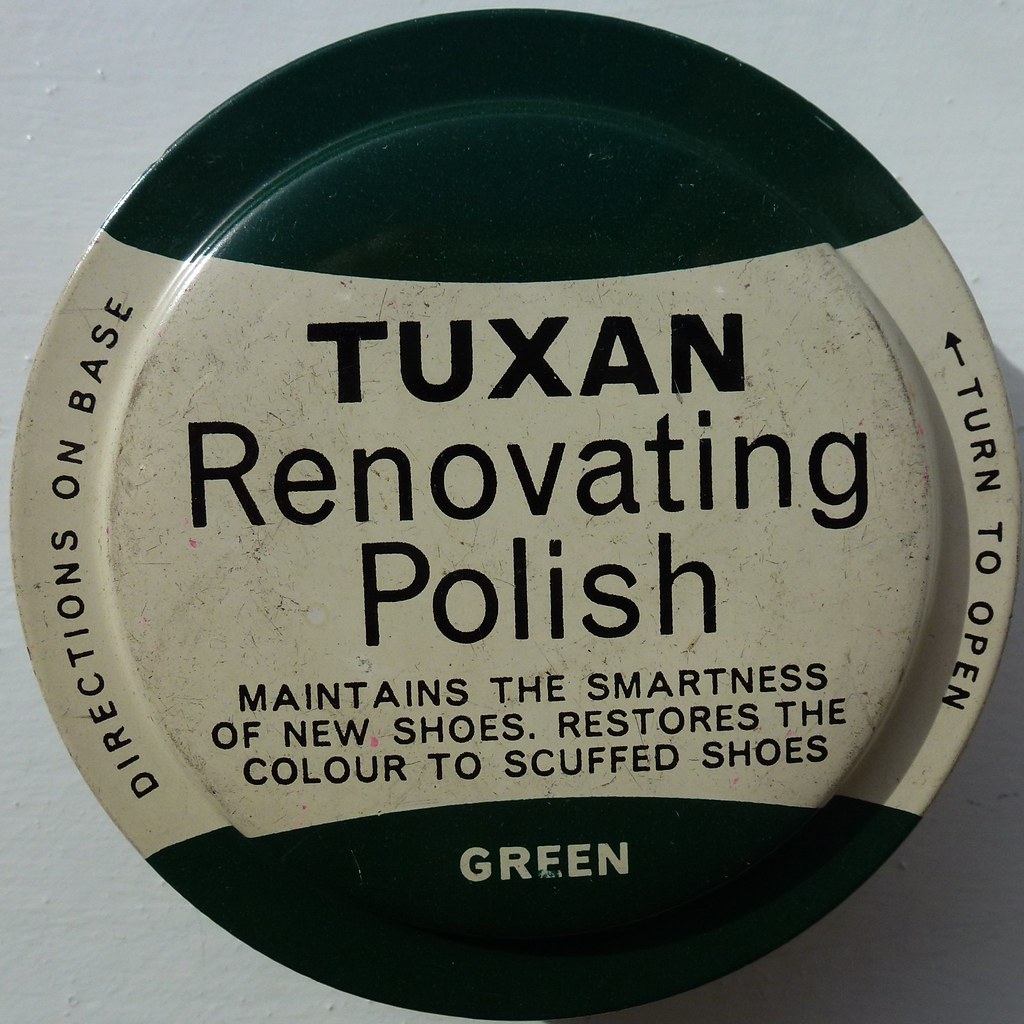This image is a detailed close-up of the top of a jar or can of shoe polish. The cap prominently features the brand name "Tuxan" in bold black letters, with the words "Renovating Polish" beneath it. It provides the slogan "maintains the smartness of new shoes, restores the colour to scuffed shoes," indicating its function. Notably, "colour" is spelled in the British manner, suggesting it might be a foreign product. The cap has a partially green top and bottom, with the word "green" in white positioned between these sections. The sides of the cap are marked with instructions: "turn to open" on the right with a small black arrow pointing up and to the left, and "directions on base" on the left. The background of the image is a light gray, with the cap having a convex shape against this backdrop.